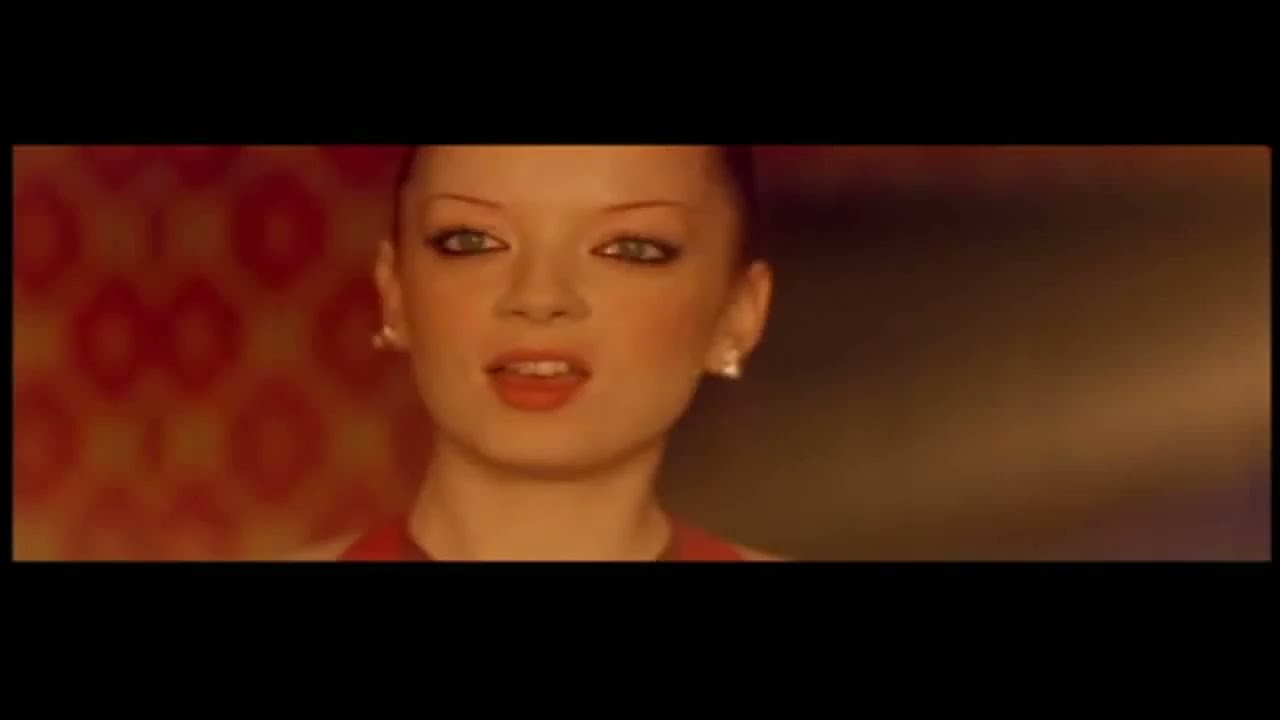The image features a young Caucasian woman, likely in her 20s, framed by a black trim at the top and bottom, with thin vertical black pinstripes along the sides. The central portion of the picture is a close-up that captures her from her forehead down to the tops of her shoulders. Her dark hair is tightly pulled back, possibly into a bun. She has sparse, brown eyebrows, heavily accentuated with pencil, and is wearing prominent black eyeliner and eyeshadow around her greenish-hued eyes. Her lips are painted with a soft red lipstick, and her mouth is slightly open, revealing the top row of her teeth and the tip of her tongue beneath. She is adorned with shiny, white stud earrings and dons a red dress that closely fits her neckline, exposing her bare shoulders. The background behind her is blurred, with shades of pink, red, and cream, featuring discernible red ovals on the left side and a mix of steel gray and brown hues on the right. The image's overall size is approximately six inches wide and three inches tall.